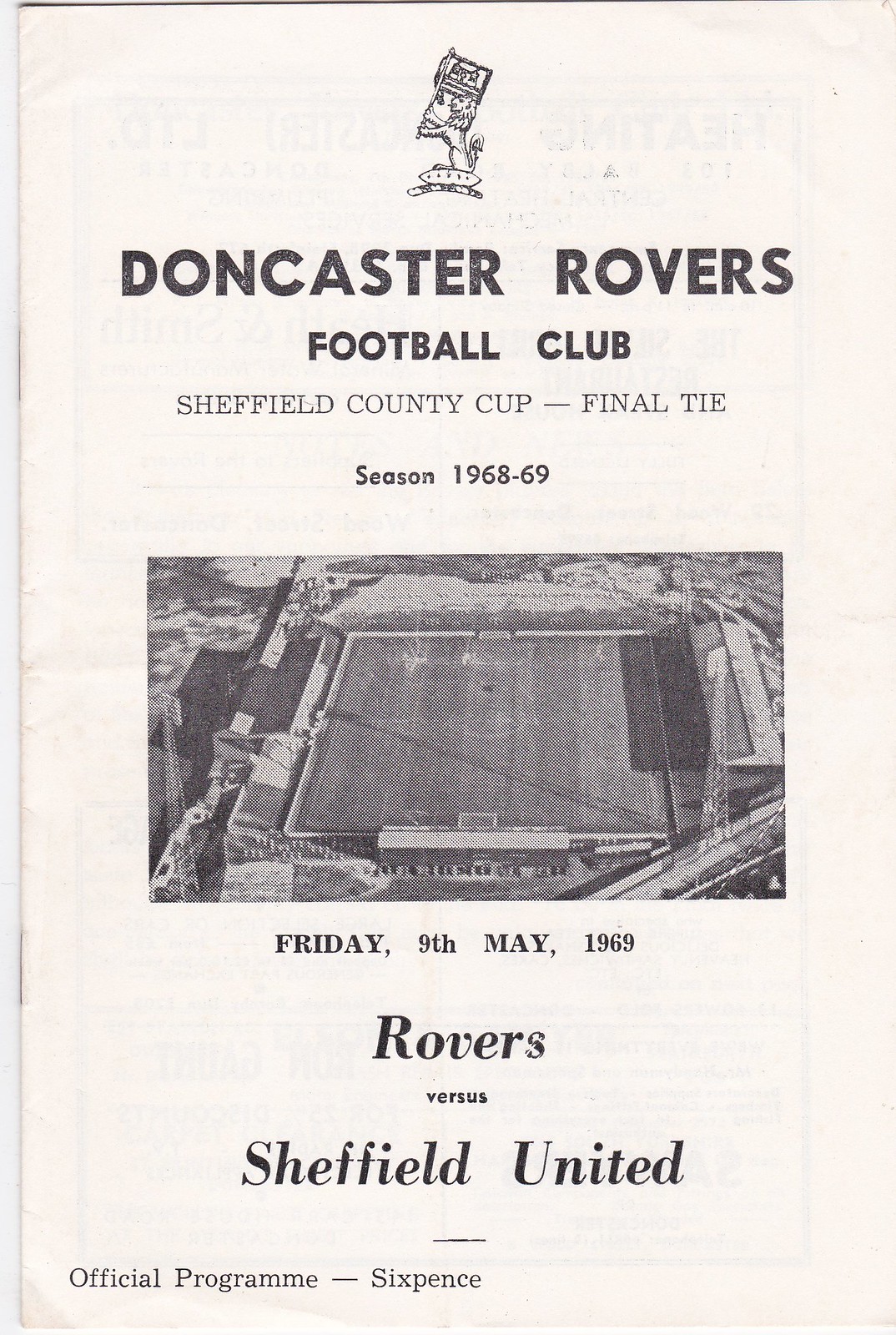This image depicts the front page of a football program for a significant match. The background is predominantly white, featuring a central black and white drawing at the very top, which somewhat resembles a head, possibly holding a surfboard, though the illustration is not clear. Directly beneath this image, in bold black letters, is the title "Doncaster Rovers Football Club". Further down in slightly lighter black letters, it reads "Sheffield County Cup Final Tie". Following this, in standard black font, the text indicates "Season 1968-69". The middle of the page showcases a grainy, black and white aerial photograph of a soccer field. Below this image, in dark black letters, the date is specified as "Friday 9th May 1969", followed by italicized text declaring "Rovers vs. Sheffield United". In the bottom left corner, the text "Official Program - Six Pence" appears in small lettering.